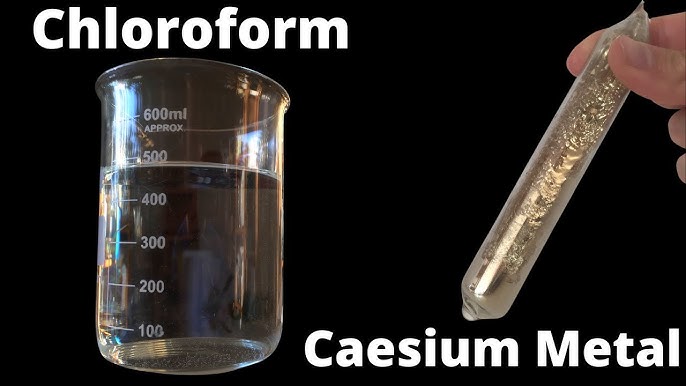The image features a black background with two main objects: a large glass beaker on the left and a test tube on the right, held by two fingers. The beaker, marked with milliliter measurements up to 600 ml, is filled with a clear liquid up to the 500 ml line and labeled "CHLOROFORM" in bold white letters at the top. On the right side, a clear cylindrical test tube, held by fingers, contains a shiny, gold-like substance. This tube is labeled "CAESIUM METAL" in bold white letters at the bottom. Both labels are prominently displayed in the same bold white text, contrasting sharply against the dark background.